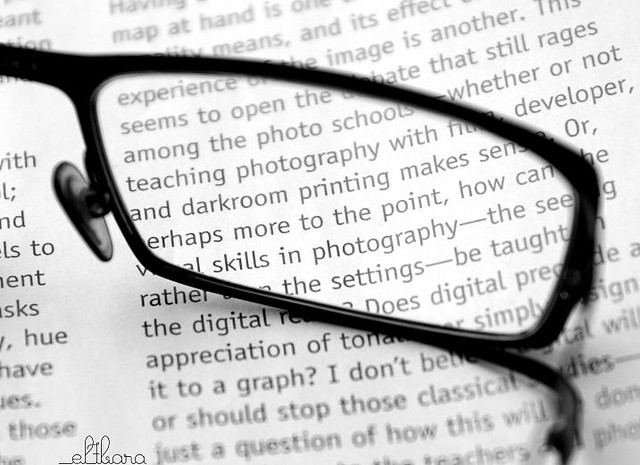This image features a detailed close-up of a single lens from a pair of glasses resting on an open page of a book. The background page is white with black text, though the text isn't clarified or altered by the lens, suggesting the glasses may lack actual lenses. The eyeglass lens holder is prominently centered in the image, with hardly any part of the frame visible. In the bottom left corner, there is a cursive signature that appears to read "Eltz Lara" or "Eltsara," though it is somewhat difficult to decipher. The overall color scheme is monochromatic, with shades of white, black, and gray. The book page contains random text fragments discussing photography, adding to the scholarly or contemplative nature of the scene. Around the edges of the photo, there is a subtle bokeh blur, highlighting the central focus on the glasses and the book page.